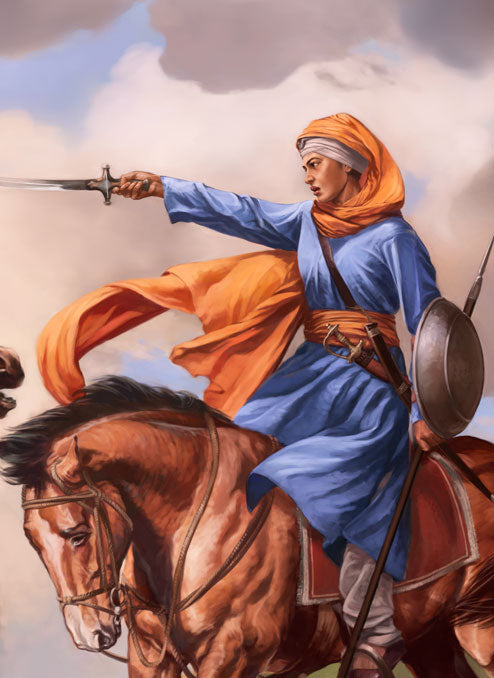The painting depicts an intricately detailed scene featuring a warrior, who appears to be an Asian woman, mounted on a light brown horse. The horse, with a black mane blowing in the wind, faces to the left with its head bent down slightly. It wears brown leather bridles and a saddle adorned with red fabric trimmed in white. The warrior sits confidently, her billowy light blue robe fluttering in the breeze, revealing white pants beneath. She is draped in an orange sash around her waist and an orange scarf around her head, the ends of which are also caught in the wind. Her feet are secured in metal stirrups, and she wears brown shoes. In her left hand, she holds a wooden spear and a silver round shield adorned on her left side. Her right arm is extended forward, holding a silver sword. A dagger in a sheath is visible on her left hip, alongside an empty brown scabbard for her sword. In the background, a mostly cloudy sky with shades of white and gray dominates the scene, with a touch of light blue peeking through the clouds in the upper left corner. The composition also includes a faint glimpse of another horse's nose on the left side of the picture, hinting at additional figures beyond the frame.